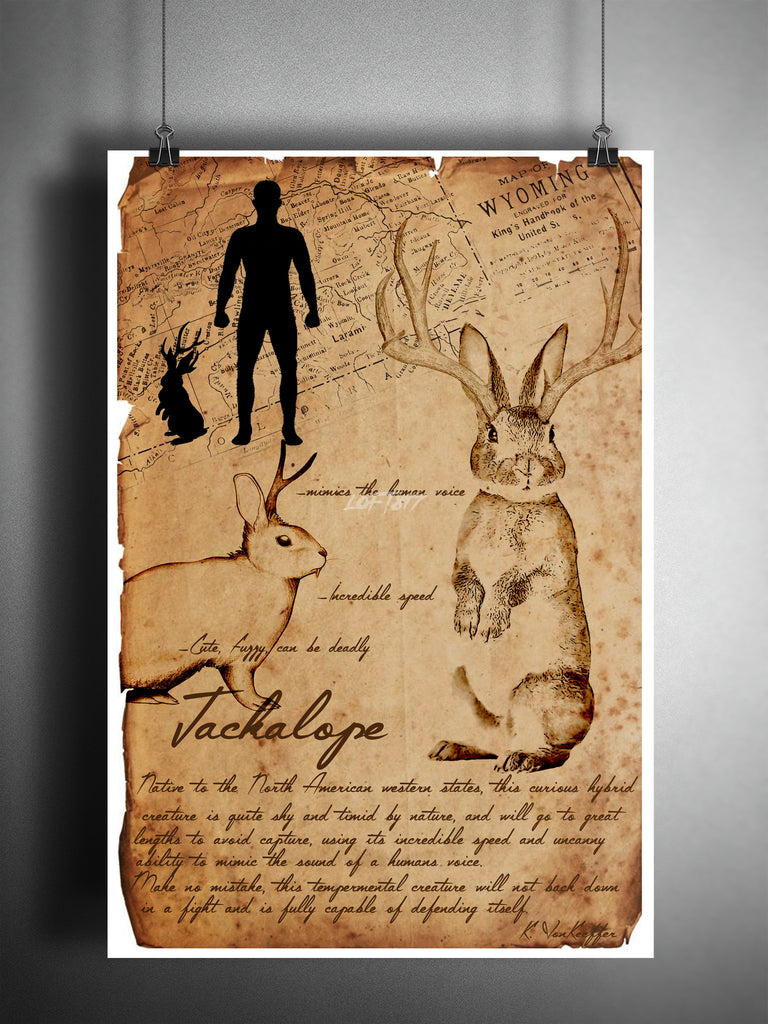The image captures an art piece suspended against a dark gray wall using wire and binder clips. The artwork itself is a print mounted on white poster board with a brown, parchment-style background designed to mimic faded newspaper, giving it an antiquated appearance. The centerpiece of the artwork features multiple illustrations and descriptions of the mythical jackalope, a fictional creature resembling a rabbit with antlers. 

At the top left of the print, there is a silhouette size comparison of a human figure standing next to a jackalope, which reaches about thigh-high. Adjacent to the human figure is a light map of Wyoming labeled "Map of Wyoming." Below this, a black silhouette of a jackalope is depicted. 

The main focus includes two detailed drawings of the jackalope: one on the left side showing its profile and the other on the right side depicting it upright on its hind legs with antlers outstretched. Between these illustrations, descriptive text extols the jackalope's traits, noting its mimicry of human voices, incredible speed, and dual nature of being both cute and potentially dangerous. Below the text, a larger cursive script reads, "Jackalope, native to the North American Western states. This curious hybrid creature is quite shy and timid by nature and will go to great lengths to avoid capture, using its incredible speed and uncanny ability to mimic the sound of a human voice. Make no mistake, this temperamental creature will not back down in a fight and is fully capable of defending itself." 

In the lower right-hand corner, the artwork is signed by "K. Von Kepher." The overall effect of the piece blends artistic whimsy with the allure of mythical folklore, giving viewers a detailed and imaginative portrayal of the legendary jackalope.